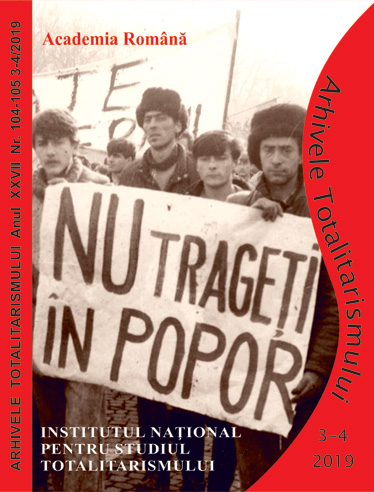The image appears to be a cover of a book with the title "Academia Romana" prominently displayed at the top. In the center, there is a black-and-white photograph of four young men who seem to be protesting, holding up a white banner with the bold black text "NU TRAGETI IN POPOR," translated as "Do not shoot at the people." 

The man on the left has dark hair and is holding one edge of the banner. The two men in the middle include one wearing a hat and a dark coat with a turtleneck, while the other has shorter, dark hair. The man on the right, also wearing a hat, holds the other edge of the banner. All four of them look visibly upset.

There are red sections on both the left and right sides of the image, with the left section featuring intricate, swirly patterns. These sections contain text related to totalitarianism, indicating this is the 27th edition of the book, and reference the date March 4, 2019 (formatted as 3-4-2019). Additionally, beneath the central photograph, there is white text that reads "Institutul National pentru Studiul Totalitarismului," which translates to "National Institute for the Study of Totalitarianism."